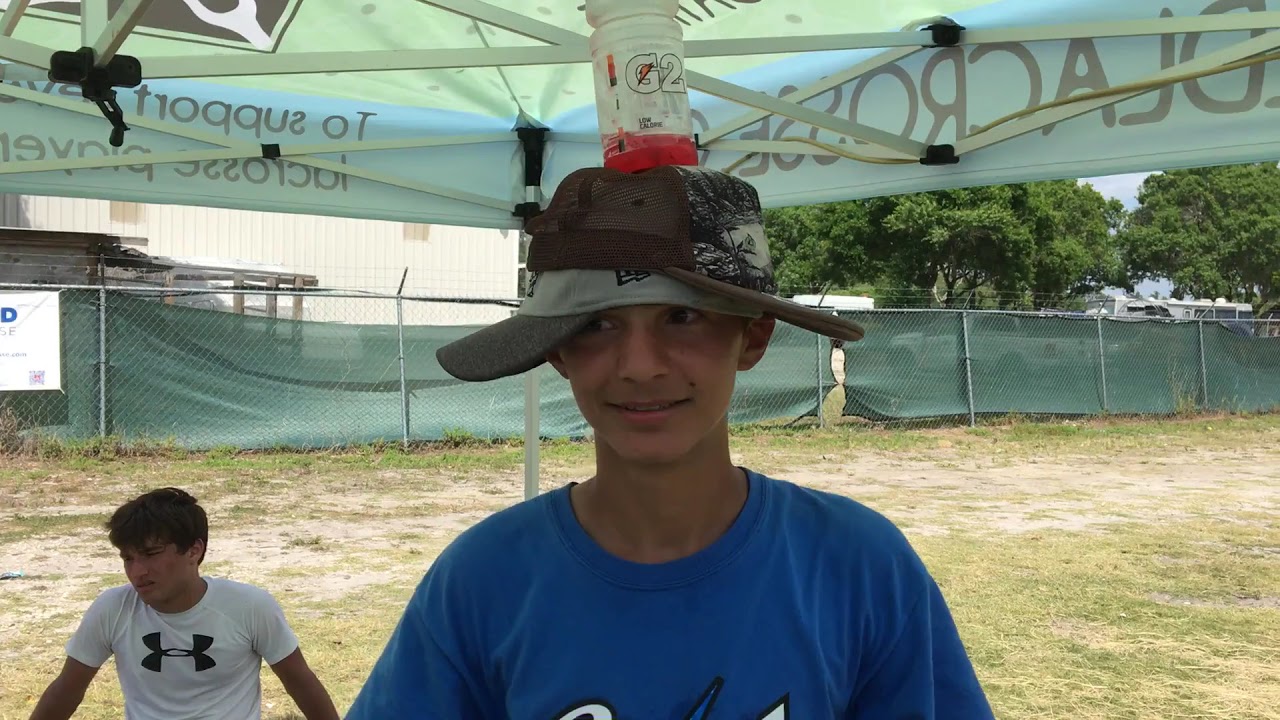In the image, a young Caucasian boy, likely aged between 10 to 14, stands under a temporary white canopy tent with a silver frame and black connecting pieces. The boy is wearing two baseball caps, each tilted sideways in opposite directions, and he balances a nearly empty red Gatorade bottle on top of them. He is dressed in a blue T-shirt and is looking to his right, away from the camera. The setting appears to be an industrial park or a less maintained field, evidenced by a barbed wire fence, industrial buildings, and vehicles like trucks or RVs in the background. The ground beneath them is a mix of dirt and sparse, patchy green grass. Near him sits another boy of the same age group, wearing a white T-shirt with a black Under Armour logo. The canopy tent has some visible text indicating it may be part of a charity event.